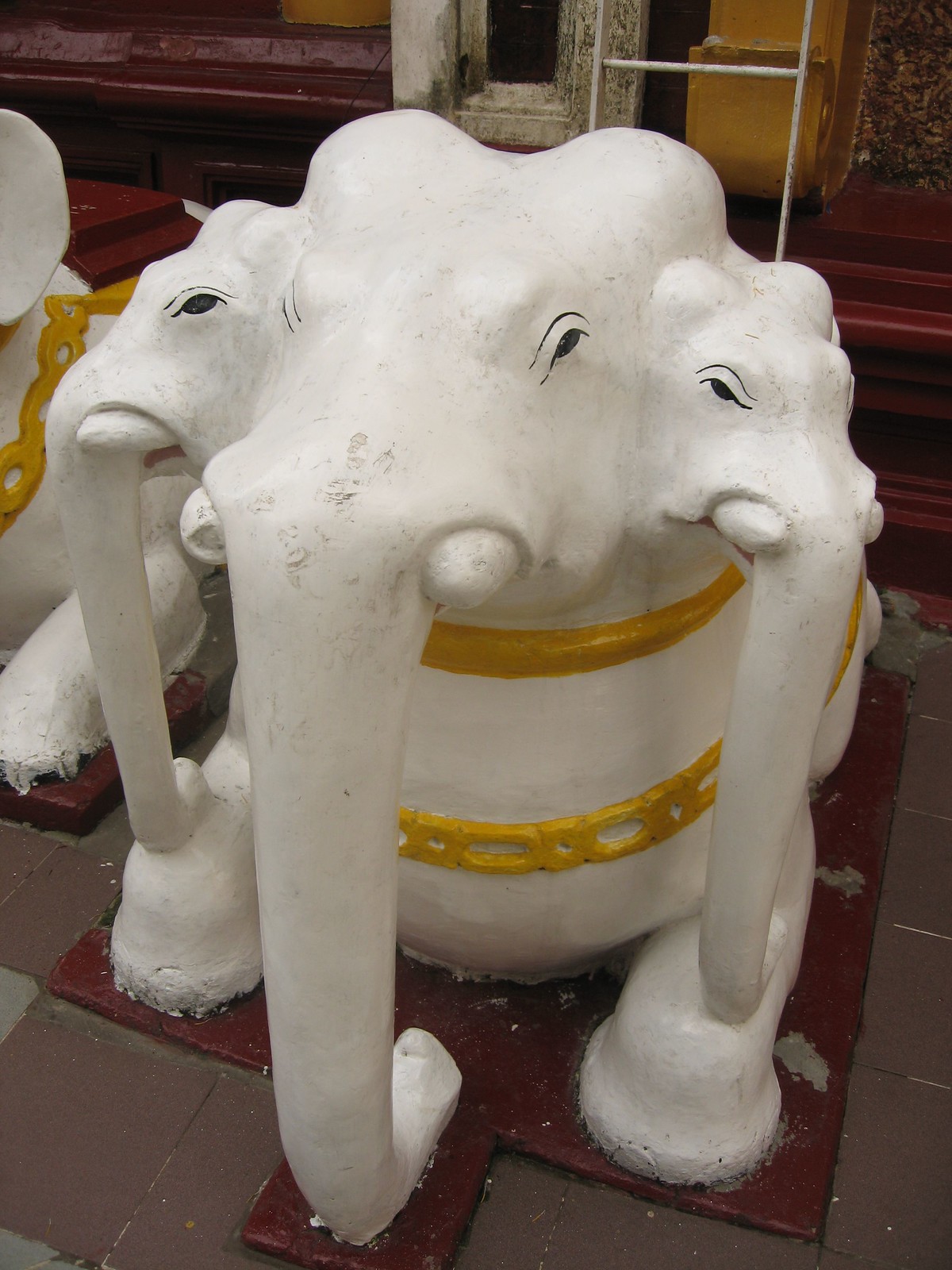This indoor photograph captures a detailed close-up of an intricate statue centered prominently in the image. The statue features a cylindrical white base adorned with yellow stripes, one of which resembles a chain. The top of the statue prominently displays a unique three-headed elephant formation. The central head faces forward, while two smaller heads extend outward where the ears would traditionally be. None of the elephant heads have tusks, and their long white trunks curve downwards, touching the ground. The elephants' eyes are black, creating a striking contrast against their white heads. The legs of the statue are also white.

The statue rests on a brown platform situated on a cobblestone ground composed of red and gray stones, with several maroon tiles accenting the area around the statue. In the background, reddish steps and a gold-hued wall add to the rich color scheme of the setting. Part of another statue is visible to the left, partially cut off due to the framing of the photo. Additionally, the background reveals a maroon-fronted building, possibly a store or temple, enhancing the indoor setting's ambiance with its brown window sills and further maroon tones. Subtle black markings on the statue suggest its age, adding historical texture to the scene.